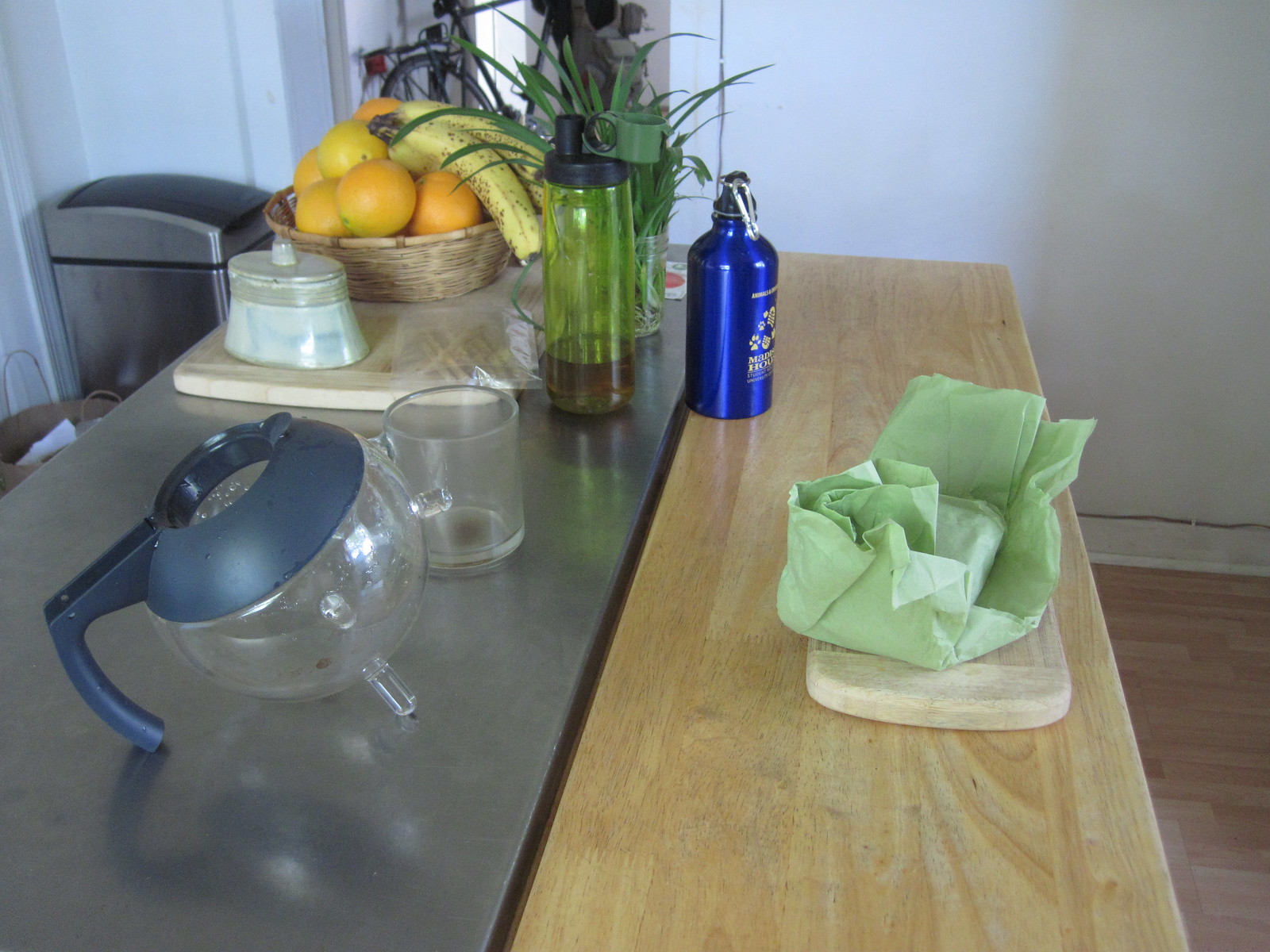The kitchen scene is an intimate and bustling area characterized by a mixture of natural and metallic elements. Dominating the view is a long, slender wooden table, likely used for breakfast, positioned adjacent to a matching-height metal surface. On the metal surface rests a spherical coffee pot, a transparent glass mug, and a striking green water bottle filled with a brown liquid, possibly tea, featuring a black lid. A wooden cutting board holds a basket of vibrant oranges with a couple of bananas perched on top, alongside a mysterious covered white dish, potentially a sugar bowl but with an unusual design.

The background reveals lush greenery, perhaps from a potted plant, contributing a fresh atmosphere to the space. On the wooden table lies a smaller cutting board and a crumpled green napkin, possibly concealing a piece of bread. An aluminum anodized water bottle with intricate patterns of white or exposed aluminum and unreadable text also sits on the table. The room is anchored by a light-colored wooden floor, white walls, and what appears to be baseboard heating. Additionally, there is a silver, covered trash can, completing the cozy yet functional kitchen environment.